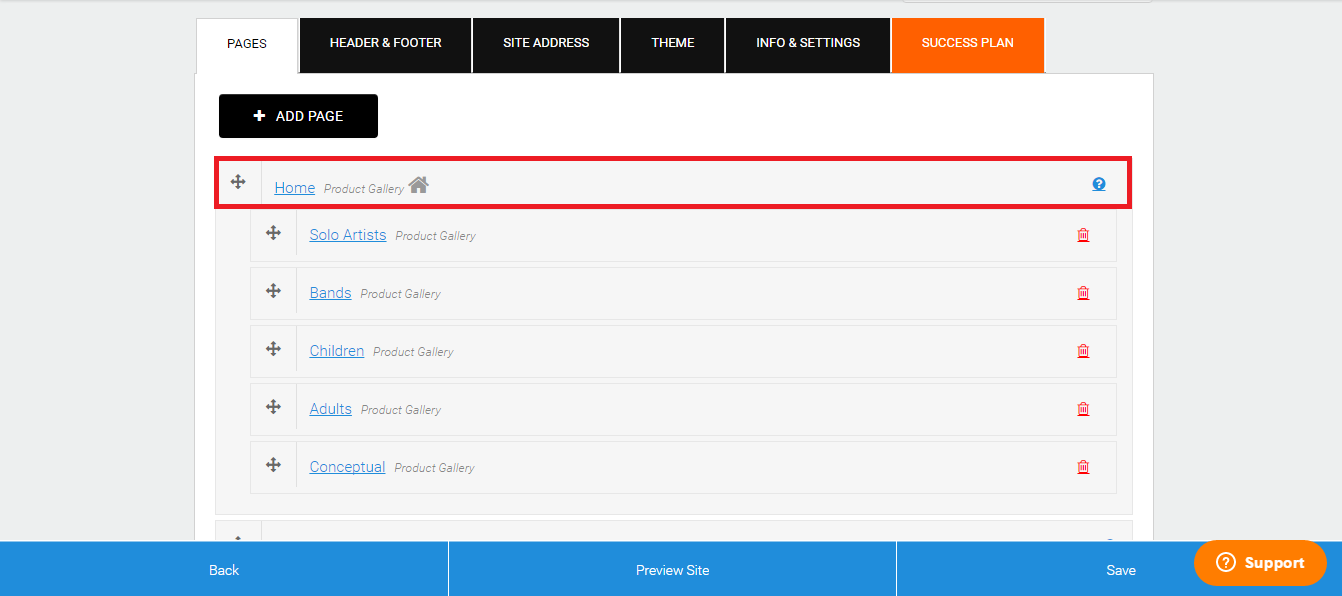Here's a detailed and cleaned-up description of the image provided:

---

The image showcases a website editor interface with a gray background. At the center is a prominent white box featuring various interactive elements and navigation tabs. At the top of the white box, there are several tabs. The first tab is labeled "Pages" in white. The subsequent tabs—"Header and Footer," "Site Address," "THFMF," "Info and Settings," and "Success Plan"—are all in black, except for the "Success Plan" tab which is highlighted in orange.

Inside the white box, there is a clear layout for managing web pages. At the top, there's a black button labeled "Add Page" with a plus sign next to it. Directly below this button, there is a search bar outlined in red. To the right of the search bar, the text "Home" is visible and underlined in blue.

Below the search bar, there are several page categories listed with corresponding actions on the right side to delete them:

- "Solo Artist" (which has a trash icon to the right)
- "Bands" (also with a trash icon on the right)
- "Children" (written and underlined in blue, with a trash icon on the right)
- "Adults" (written and underlined in blue, with a trash icon on the right)
- "Conceptual" (written and underlined in blue, with a red trash icon on the right)

At the bottom of the white box, there are two important buttons: "Preview Site" and "Save." Additionally, next to the "Save" button, there's a notable circular oval button with the text "Support" inside it and a question mark enclosed within a circle.

---

This enhanced caption provides a clear and concise description of the image, making it easy to visualize the website editor interface.